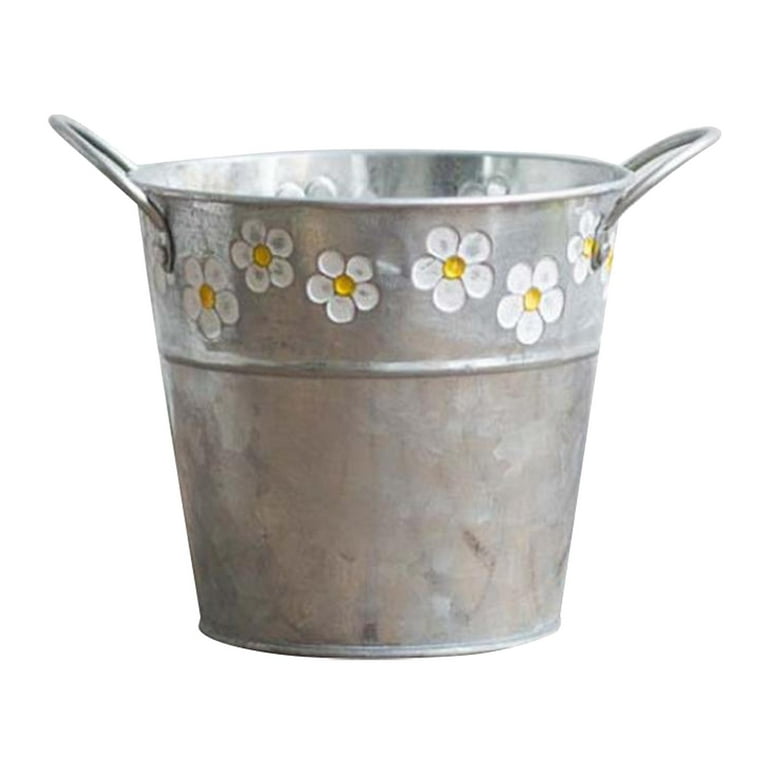The image is a full-color close-up photograph featuring a silver aluminum bucket centered against a plain white background. The bucket, which stands about a foot tall, has a cylindrical shape that slightly widens toward the top. It features two metal hooped handles, one on each side, arching over like semi-circles and secured with bolts. Two ridges encircle the bucket: one near the top edge and one just above the center. Painted onto the bucket, near the top, is a decorative row of daisies—each flower showcasing five white petals and a yellow center—arranged in a curvy line that wraps around the entire circumference. Additionally, there are minor smudge marks and fingerprints visible on the bucket's surface, adding a touch of rustic charm. The background is purely the white of the screen, highlighting the bucket as the focal point. The daisy pattern appears both on the outside and slightly inside the bucket, suggesting a consistent decorative theme.